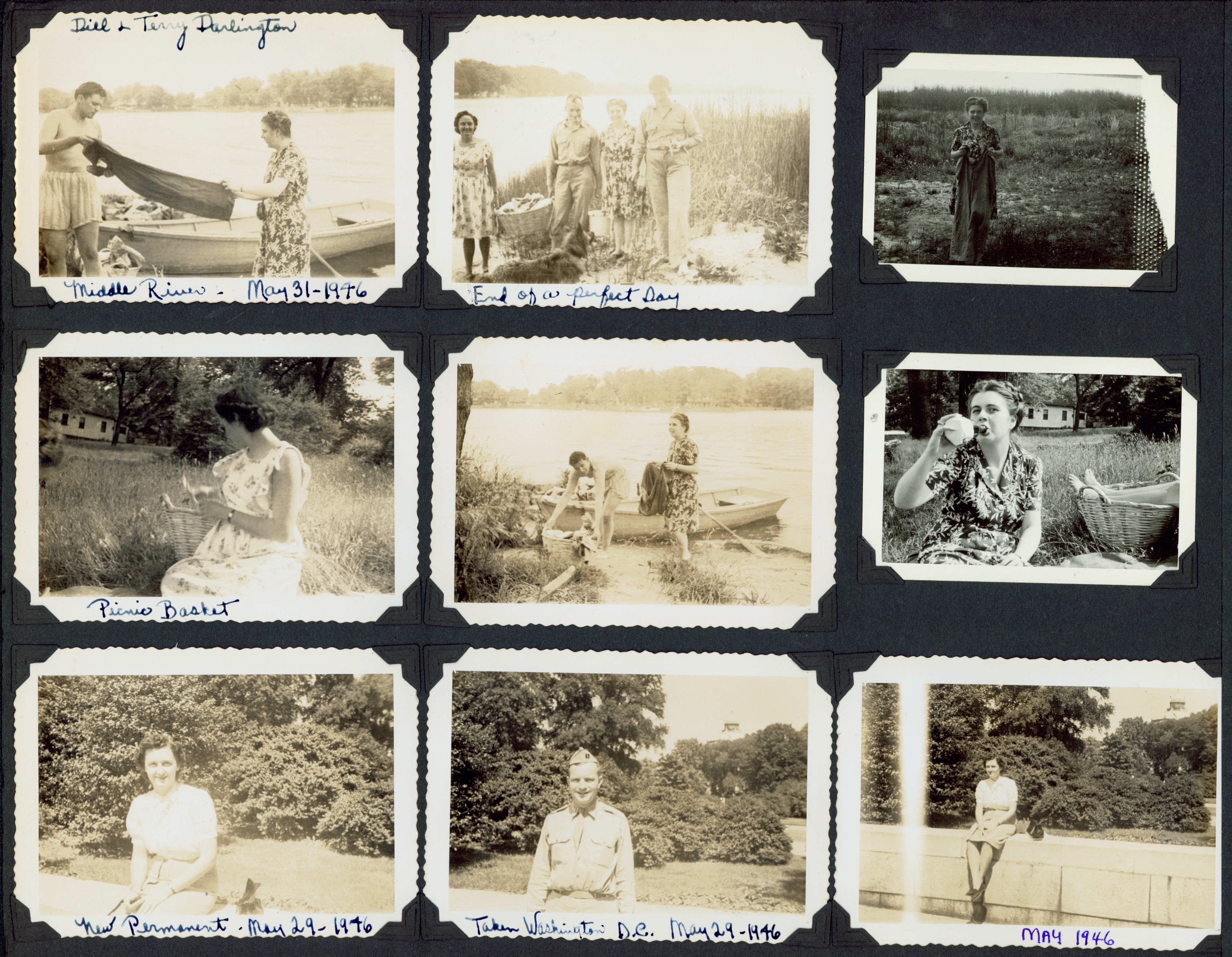This photo album page showcases nine black-and-white photographs from 1946, meticulously arranged on a vintage black construction paper page common in the scrapbooks of the 1940s and 1950s. Each photograph is secured with adhesive corner mounts and is accompanied by handwritten captions, although some handwriting is difficult to decipher. The pictures are organized in three rows of three, capturing moments primarily featuring women, with themes of canoeing, picnicking, and outdoor leisure activities.

In the top-left photo, labeled "Dill and Terry Darrington, Middle River, May 30th, 1946," a man and woman stand in front of a canoe near a lake, folding a dark object—possibly a blanket or article of clothing. The top-middle photo, captioned "End of a Perfect Day," shows four people standing near a river, two of whom hold a large basket that presumably contains fish. The top-right photo features a woman standing in a field, wearing a dress, with trees in the background.

The middle row begins with a photo titled "Picnic Basket," depicting a woman in a sleeveless summer dress looking away from the camera. The middle photo in this row shows two people in front of a canoe by a river, and the rightmost photo captures a woman drinking from a bottle while another person’s feet rest in a picnic basket behind her.

In the bottom row, the left photo labeled "New Permanent, May 29th, 1946," displays a woman with freshly styled hair sitting in front of bushes. The middle photo, captioned "Taken, Washington, D.C., May 29th, 1946," features a man in an army uniform. The final photo, dated May 1946, shows a woman sitting on a ledge with bushes behind her.

This meticulously arranged page not only preserves these precious memories but also provides a nostalgic glimpse into the leisurely activities and fashions of the mid-20th century.